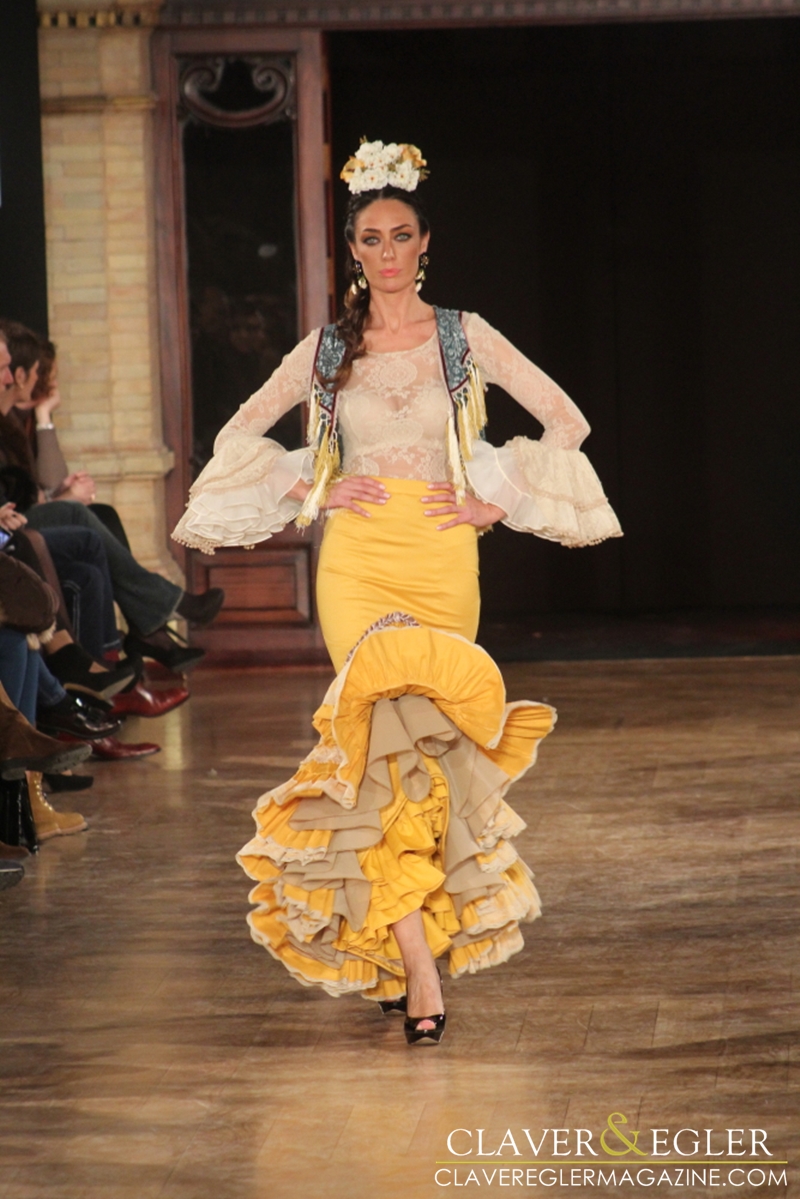The highly detailed photorealistic image captures a striking scene from a fashion show runway. A woman with light skin and dark hair, which is styled up and draped over her left shoulder, confidently walks the runway with her hands on her hips. She is adorned with a headpiece made of yellow and white flower-like shapes that complement her elegant hairstyle. Her ensemble features a delicate, white see-through lace top with floral designs, revealing a white bralette underneath. The top also boasts billowy sleeves that flare around her wrists. Adding to the layered texture of her outfit, she wears a fringed vest in shades of blue and yellow over the lace top. 

Her lower half is highlighted by a form-fitting yellow skirt that flares out at the bottom, showcasing an intricate cascade of yellow, brown, and white ruffles reminiscent of a flamenco dancer’s attire. She completes the look with black heels. The patterned brown marble or stone floor beneath her adds a touch of sophistication to the scene. 

In the background, a mix of black walls, wooden elements, and a golden brick post or column can be seen, along with silhouettes of seated attendees, their crossed legs hinting at their attentiveness. The image is branded with the words "Claver and Eggler" in white and gold lettering, and below that, "ClaverEgglerMagazine.com" is printed in smaller letters in the bottom right-hand corner.